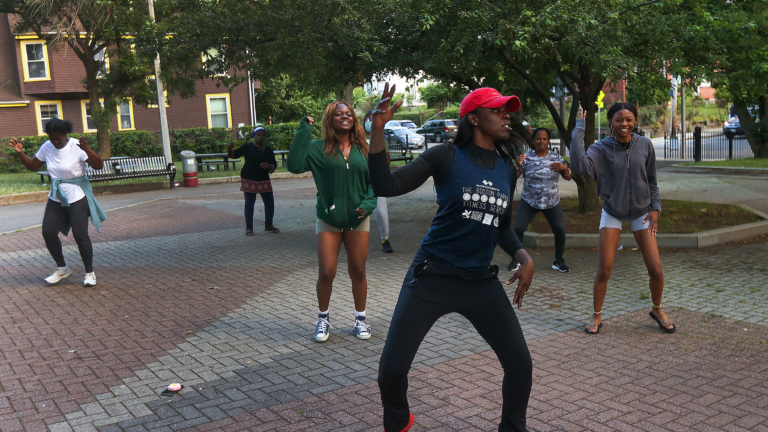The image showcases an outdoor setting where seven African American women are dancing together. They seem to be in a park, as suggested by the presence of surrounding trees and a concrete ground. One woman, distinguishable by her red hat, blue shirt, black jeans, and red shoes, appears to be leading the group in a coordinated dance routine. The women are dressed comfortably in a variety of colorful attire, including black, white, green, military gray, and patterned clothing. In the background, there's a prominent brown building with yellow windows, and a section of a black fence can be seen in the top right corner. Additionally, there are cars visible in the distance and a park bench nearby, enhancing the sense of an open, communal space. The scene captures the energetic and communal spirit of the group as they follow along to a song or dance coordination, adding vibrancy to the park setting.